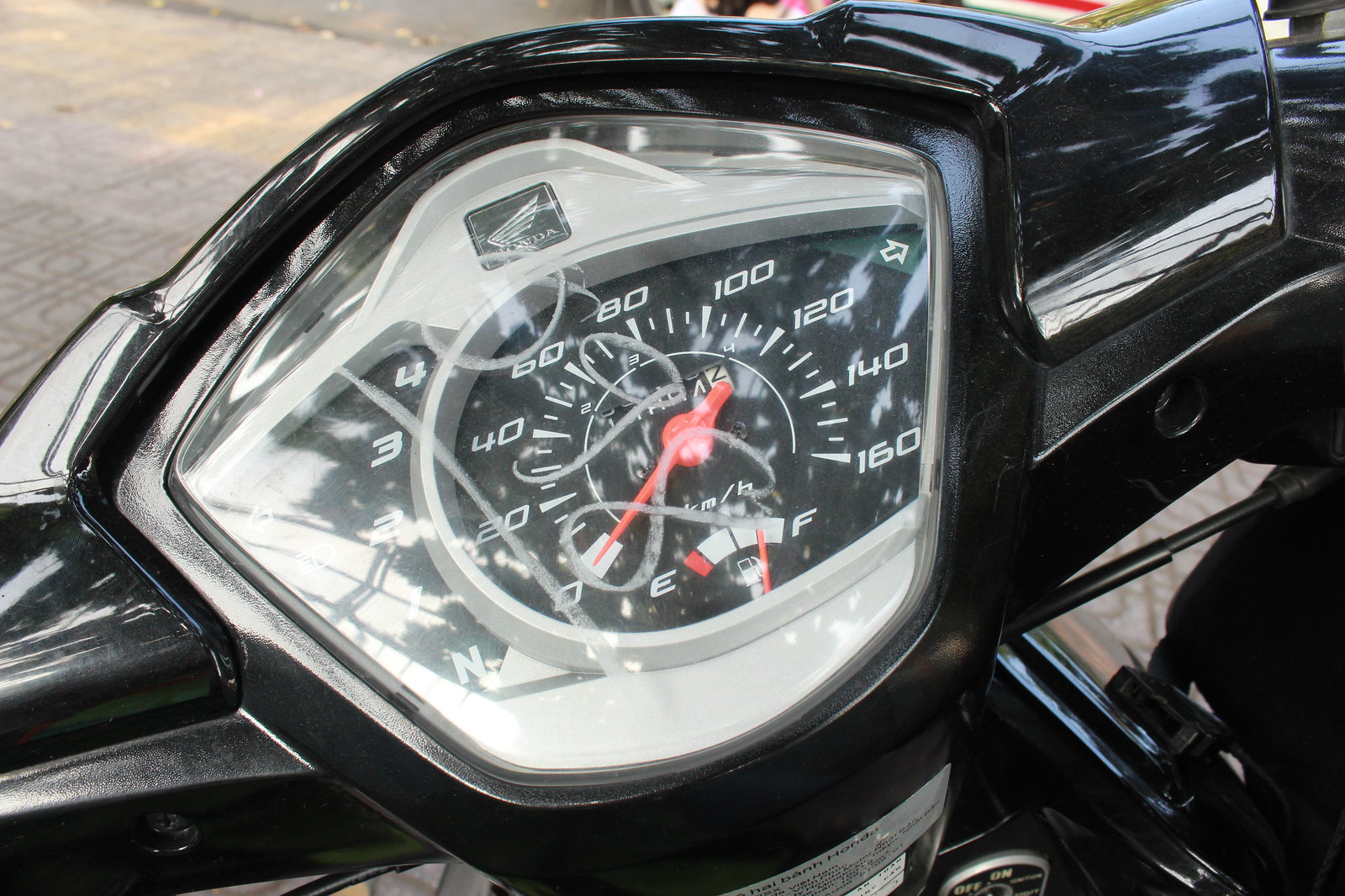The image features the odometer of a Honda motorcycle, prominently displaying the iconic Honda logo at its center. The logo is encapsulated in a black square with the white letters "HONDA." There is a slight smudge on the odometer screen. The odometer's dial is black with white numbers arranged in a half-circle, ranging from 0 to 160. The needle, which indicates the speed, is red. Surrounding the odometer is an all-black side panel, which exhibits a noticeable glare, adding a reflective sheen to the overall composition.

In the background, the photograph reveals an outdoor setting. A sidewalk occupies the top left corner, strewn with golden-colored leaves, suggesting an autumnal scene. The sidewalk itself is light gray, contrasting with the darker elements of the motorcycle's dashboard. The image captures not only the intricate details of the motorcycle's odometer but also hints at the serene outdoor environment in which the photograph was taken.